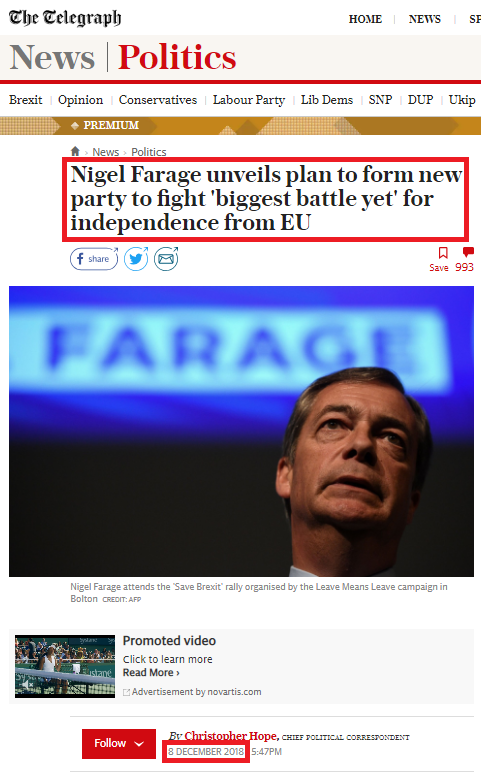This is a detailed descriptive caption for the provided screenshot:

---

Screenshot of The Telegraph's website displaying a news article about Nigel Farage. The page features a large font header with the word "News" in gray and "Politics" in red. The name of the website and newspaper, "The Telegraph," is prominently positioned in the top-left corner. On the right-hand side of the page is a photograph of Nigel Farage, depicted looking upwards into the air. The majority of the page has a white background. In the bottom-left corner is a red follow button. The main article on display is enclosed within a red box and is titled "Nigel Farage unveils plan to form new party to fight biggest battle yet for independence from the EU."

---

This caption encompasses all the details provided and offers a clear and precise description of the image.